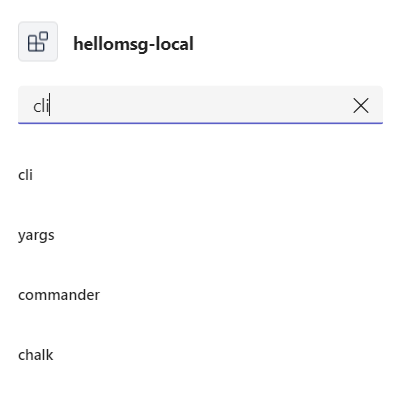This digital screenshot features a user interface with a prominent gray logo on the left. The logo consists of a square containing four smaller squares with blue shading; three of these small squares are connected, while the fourth is slightly apart but nearby. Adjacent to the logo is the bold, black text "hello msg-local." To the right of this text is a partially populated search bar with the input "CLI," accompanied by a small 'X' icon for clearing the input. Below the search bar stretches a long, straight blue line, spanning approximately five inches. Further down, there are several partially visible words, including "CLI," "yargs" (spelled Y-A-R-G-S), "commander," and "chalk."